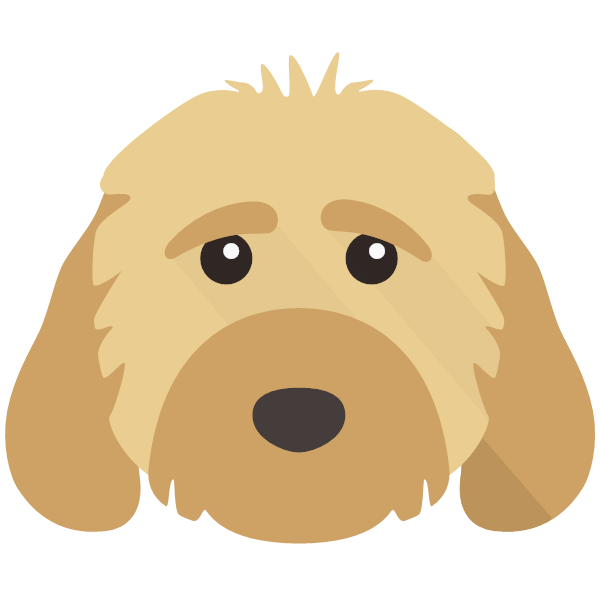This is a minimalist, cartoonish digital graphic of a dog's head set against a white background. The dog's head is primarily light tan with darker brown, floppy ears. The muzzle, also in darker brown, matches the ears and eyebrows, which are similarly dark brown. The dog’s eyes are black circles with white pupils, giving them a reflective appearance. It has a small, almost black nose and small tufts of hair sticking up from the top of its head. The depiction suggests the dog might be a small breed, possibly reminiscent of a terrier, and the overall style is quite simplified yet expressive.